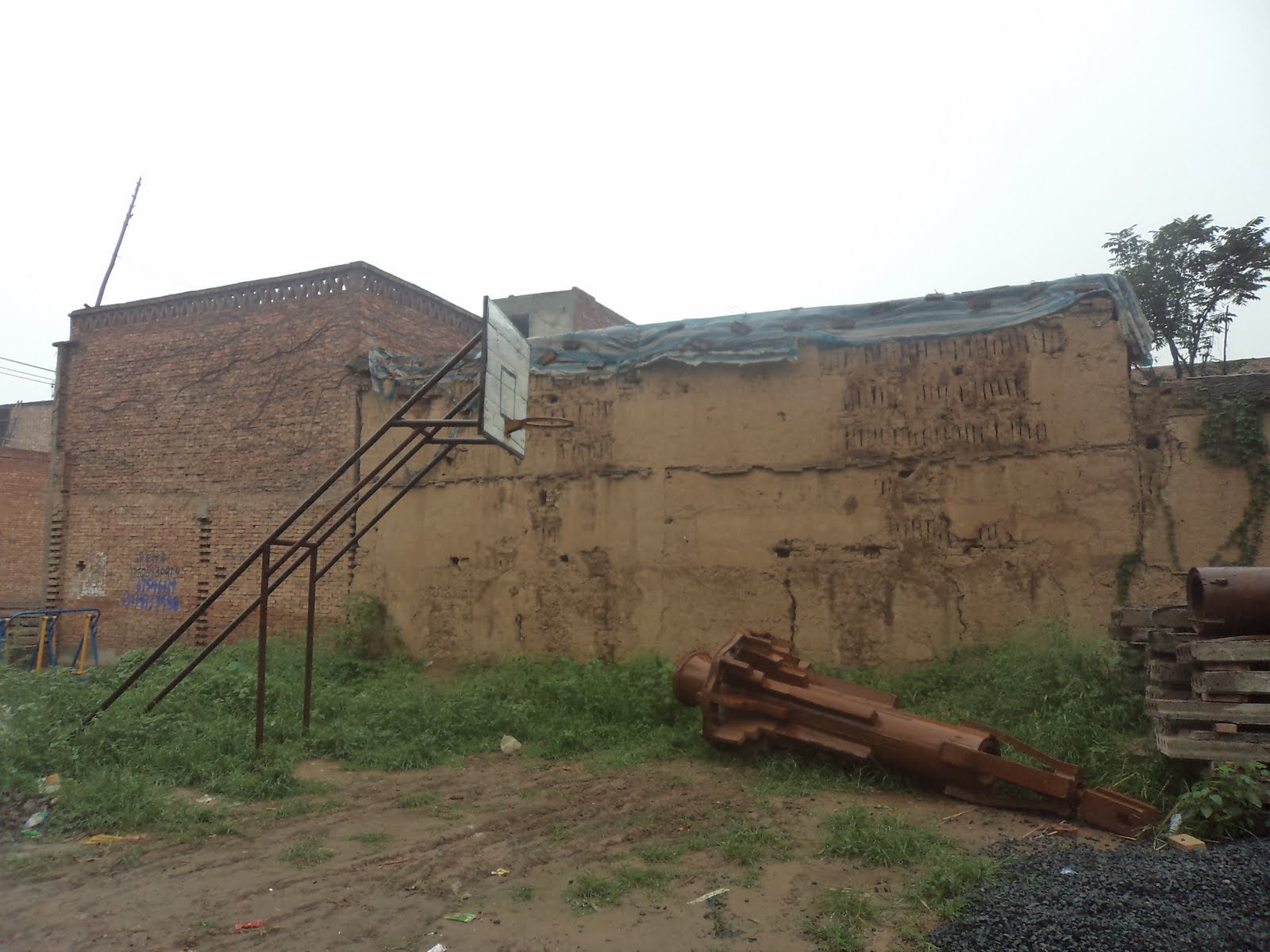The photograph captures an abandoned play area, characterized by a grassy perimeter surrounding a central sandy region. Dominating the sandy center is a large, copper-colored piece of heavy machinery, possibly from a crane, showing visible signs of decay and neglect. Adjacent to this derelict equipment, a weathered basketball hoop stands as a testament to the area’s former recreational purpose. Behind the scene, a building with a cloth roof looms, with a wooden pallet lying in front of it, further enhancing the sense of abandonment. The uneven ground hints at the once active but now forgotten place where children might have played.